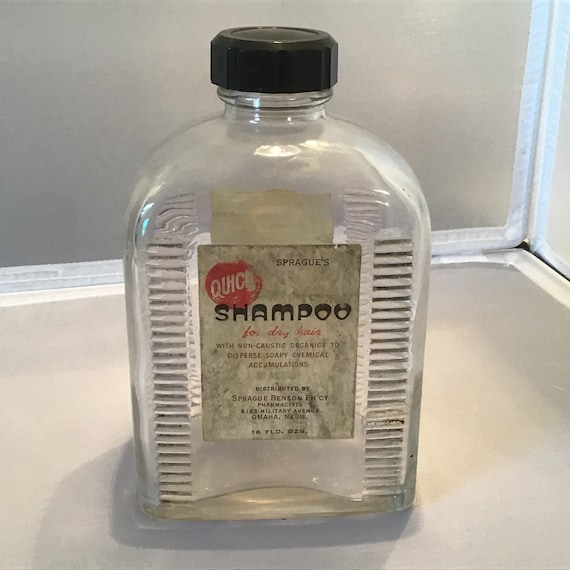The image depicts an empty bottle of shampoo with a black screw lid, likely made of glass or plastic. The bottle, which appears old and possibly decades old, has a round shape with ridges on the left, right, and back. The label, which looks like it was once white but is now quite dirty, features a red circle on the left side with unclear text that could read "Q-I-H-C" or "Q-U-H-C." The brand name "Spriggs" or "Spragues" is prominently displayed at the top. Below that, in large black letters, is the word "Shampoo," followed by the phrase "for dry hair" in red text. The label also states, "with non-caustic organics to disperse soapy chemical accumulations." Further down, in black text, it reads, "distributed by Sprigg Benson Pharmacy, pharmacists, Omaha, Nebraska," and the bottle contains "16 FLD. OZS." The setting appears to be indoors, with a translucent grey and white-bordered background, possibly resembling a folding shelf.